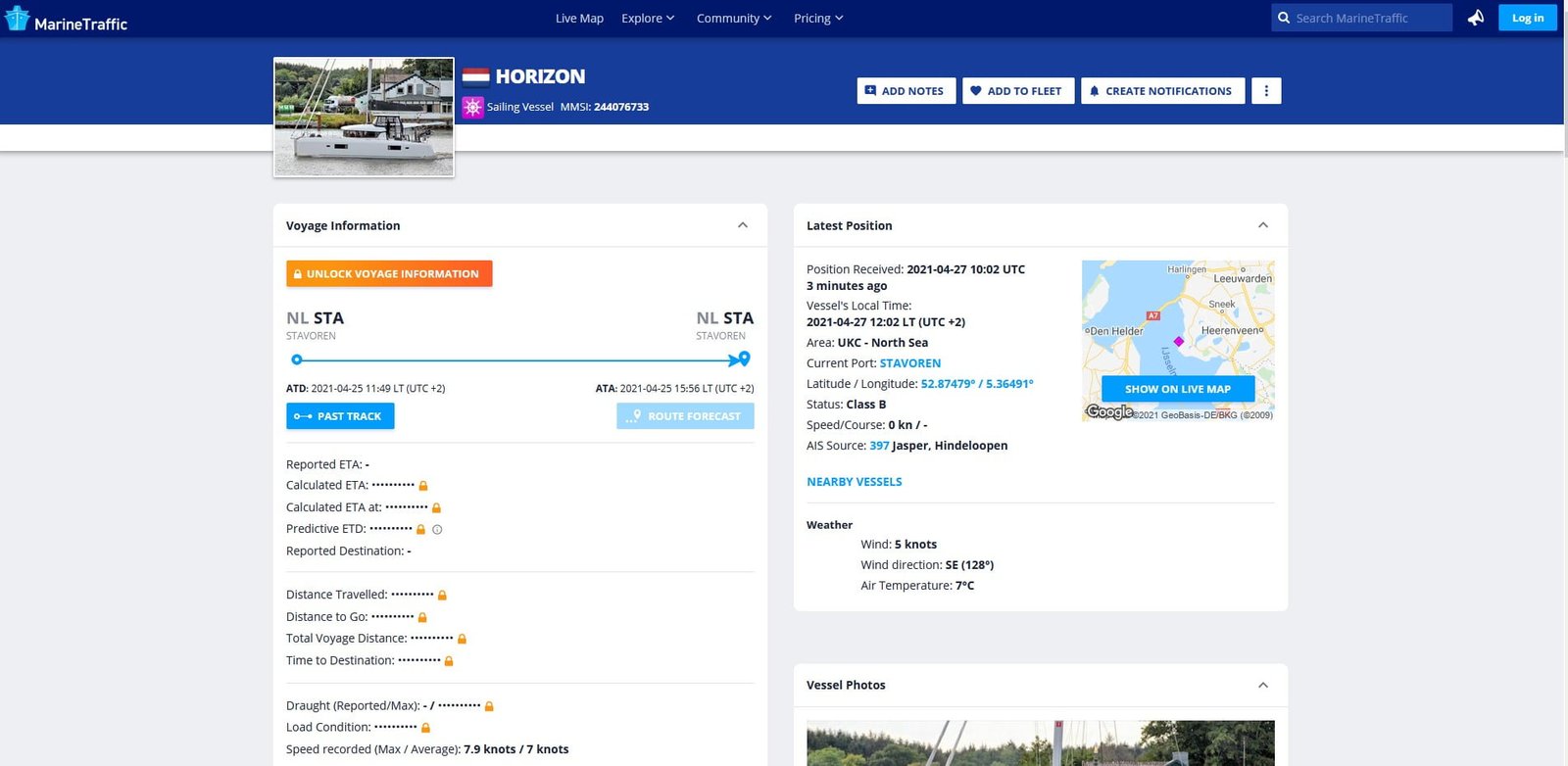This detailed color screenshot from the Marine Traffic website provides extensive information about a vessel named Horizon. 

At the top left, a blue ship icon accompanies the Marine Traffic logo. Adjacent to this, on the dark blue navigation banner, are links labeled "Live Map," "Explore," "Community," "Pricing," along with a search bar titled "Search Marine Traffic" and options to "Log In."

Below this is a lighter blue banner featuring a photograph of a white boat sailing on calm waters with hills and a white two-story building in the background. A French flag is displayed next to the vessel's name, "Horizon," identified as a sailing vessel with MMSI 244076733. Options available include "Add Notes," "Add to Fleet," and "Create Notifications."

Under the ship's photo, the Voyage Information section includes details such as NLSTA (Stavoren) with dates and times: ATD (Actual Time of Departure) on 2021-04-25 at 1149 LT (UTC+2) and ATA (Actual Time of Arrival) on 2021-04-25 at 1556 LT (UTC+2). Other data points listed include Past Track, Route Forecast, Reported ETA, Calculated ETA, Predictive ETD, Reported Destination, Distance Traveled, Distance to Go, Total Voyage Distance, Time to Destination, Drought Reported, Maximum Load Condition, with recorded speeds of 7.9 knots max and 7 knots average.

On the right side, under the Latest Position section, it notes the position was received on 2021-04-27 at 1002 UTC, 3 minutes ago, with the vessel's local time being 1202 LT (UTC+2). The area is identified as UKC-NC with the current port listed as Stavoren. The coordinates are 52.87479° N / 5.36491° E. The vessel's status is Class B with a speed/course of 0 knots and AIS source 397 from Jasper Hindalupin.

A map to the right provides options to "Show on Live Map," view on Google Maps, check Nearby Vessels, and access Weather data including wind at 5 knots coming from the SE at 28°, and an air temperature of 7°C. Below this, a partially cut-off photo is displayed in the Vessel Photos section.